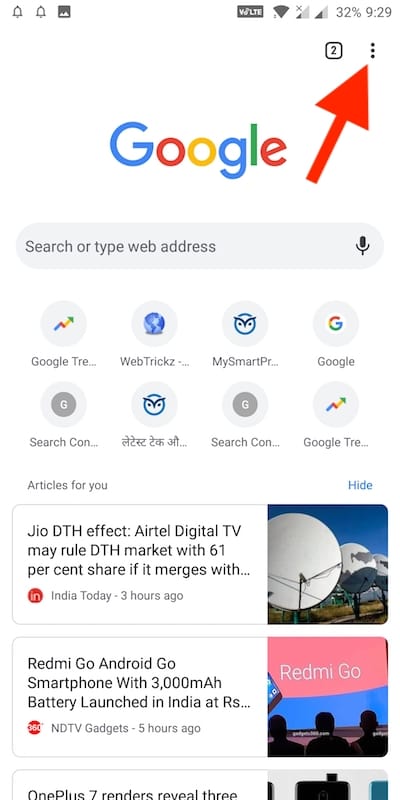The image depicts a Google Chrome browser interface with various elements highlighted for instructional purposes. 

- At the top right corner of the page, there's a blue arrow pointing to the settings button, represented by three vertical dots. 
- Below this, the address bar displays "Search or type web address" with an option for voice search.
- The bookmark bar includes several saved sites: "Google Trends," "WebTricks" (with a "z"), "MySmart... something," and a "Google" button.
- Further down, the bookmarks show "Search CON" and a Japanese site with a similar icon to "MySmart."
- Below the bookmarks, there's a section titled "Articles for You," with the option to hide this section on the right side.
- Two featured articles are visible:
  1. "Geo DTH Effect: Airtel Digital TV May Rule DTH Market with 61% Share if it Merges," from India Today, posted three hours ago. This article is accompanied by an image of large satellite dishes.
  2. "Redmi Go Android Go Smartphone with 3,000mAh Battery Launched in India," from NDTV Gadgets, posted five hours ago. The article includes an image of a group of people viewing a PowerPoint presentation about the Redmi Go smartphone.
- At the top right of the interface, there are two alert icons, an image snippet, and indicators for Wi-Fi connectivity at 32% and a battery life display. The current time is shown as 9:29.